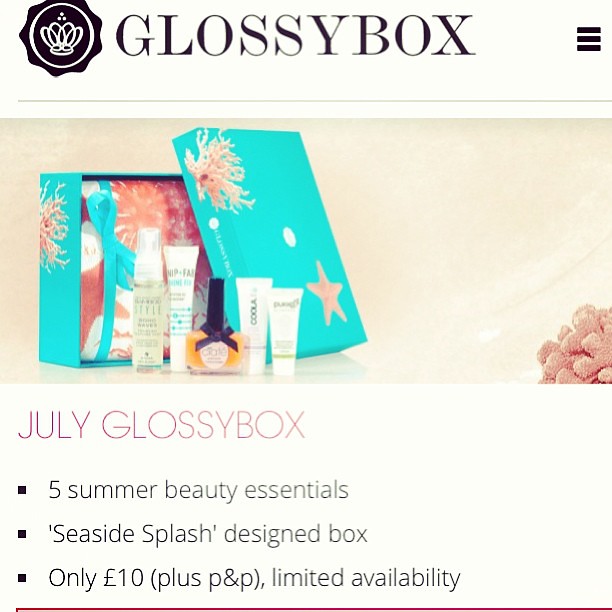This screenshot captures a mobile version of an advertisement for Glossy Box, showcasing their July edition. The top left features the company's elegant logo—a white crown within a black circular emblem, surrounded by a white circle—and the brand name "Glossy Box" in classical typography. Adjacent to this is a menu icon, indicative of a dropdown menu.

The central image displays an open gift box, designed with a seaside splash theme. The box, colored in aqua or turquoise, is adorned with illustrations of starfish, seashells, and coral, set against a light tan background that includes pink coral accents in the lower right corner.

Inside the box, there are five summer beauty essentials, including skincare products, creams, and sprays, arranged neatly. Below the image, prominent text details the key offerings: "July Glossy Box," followed by bullet points highlighting "Five summer beauty essentials," "Seaside Splash design box," and "Only £10 plus P&P, limited availability." A red line runs across the bottom of the image, visually separating this segment from any potential further content. This advertisement suggests that Glossy Box is a subscription service, likely appealing to women, delivering curated beauty products monthly.